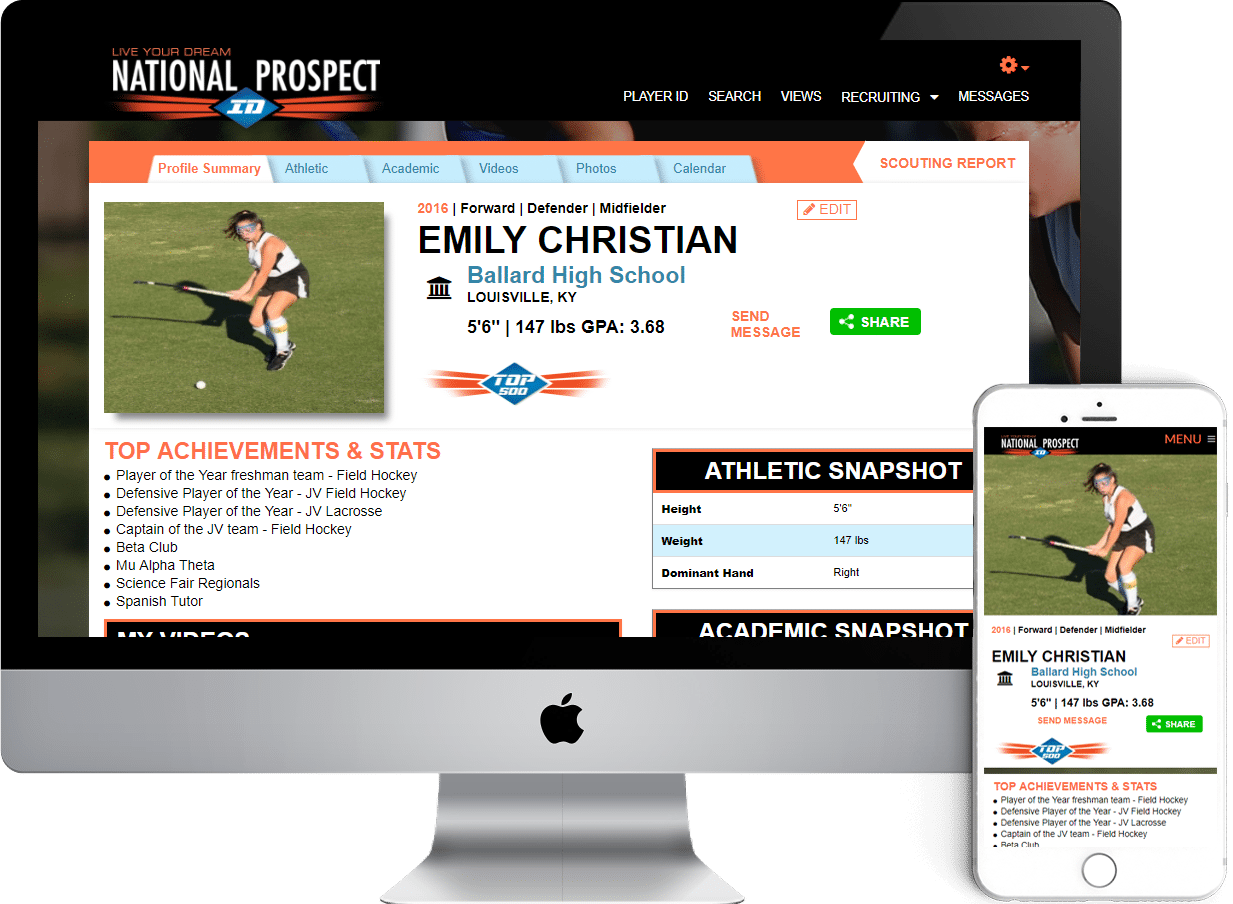The image features an Apple monitor with a silver bezel and matching stand, prominently displayed on a desk. In front of the monitor is an Apple iPhone, both screens mirroring the same content. The monitor screen showcases a mock website titled "National Prospect" emblazoned in a white font within a black rectangle at the top. Adjacent to the title, there are navigation links labeled "Player ID," "Search Views," and "Recruiting Messages."

Below the title bar, a blue diamond icon with the letters "ID" in white font is visible. This icon is accentuated by red horizontal lines radiating from its sides. Beneath this icon, a white square profile card is displayed. The profile features a high school student named Emily Christian, who attends Ballard High School in Louisville, Kentucky. Further details include her height of 5'6", weight of 147 pounds, and a GPA of 3.68.